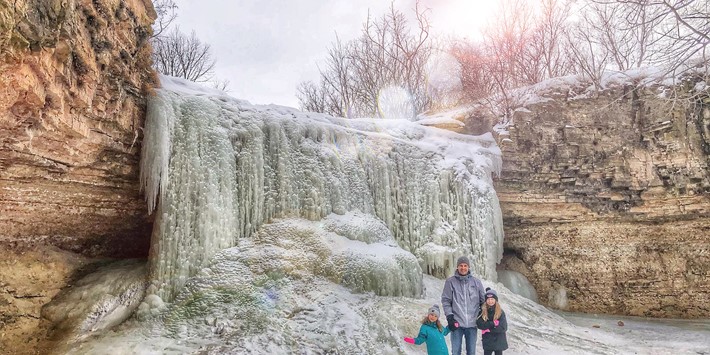In this stunning winter photograph, a father and his two daughters stand hand in hand, smiling warmly for the camera. The father, dressed in a gray jacket, gloves, and a hooded hat, is flanked by his daughters, one in a blue jacket and pink gloves, and the other in a black jacket with a fur-trimmed collar. All three don knit caps to fend off the cold. They are depicted as small figures against the majestic backdrop of a frozen waterfall, which spans approximately 20 to 30 yards across and towers about 20 feet high. The waterfall, completely frozen into intricate icicles, is framed by rugged, reddish-brown cliffs on either side. Above the cliffs and waterfall, a stark forest of bare, leafless deciduous trees reaches up to a gray winter sky. The sun, positioned around one o'clock, casts a few light flares across the image, highlighting the serene yet chilly beauty of this natural scene.